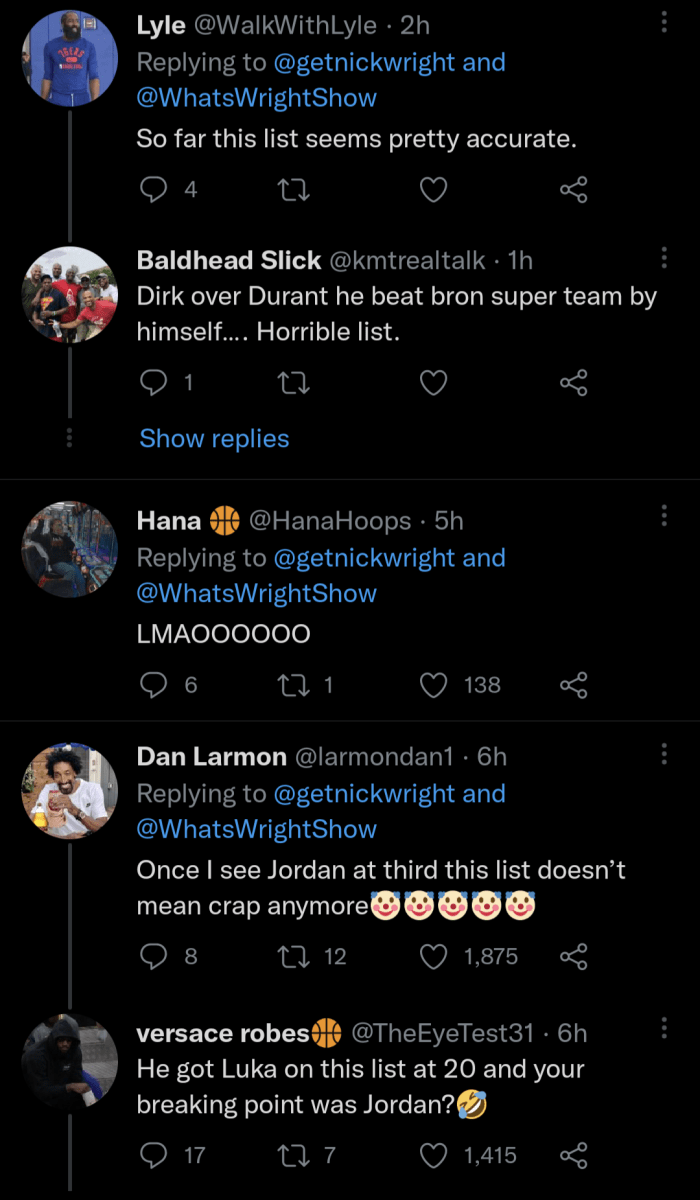Here is a detailed and cleaned-up caption for the described image:

---

This image is a screenshot of a Twitter page featuring a series of comments in response to a post by the users @GetNickRight and @WhatRightShow. The first comment is from Lyle (@WorkWithLyle), posted two hours ago, stating, "So far, this list seems pretty accurate." This comment has four replies.

The second comment is from BaldHeadSleek (@KMTrailTalk), posted one hour ago, critiquing the list: "Derek over Durant? He beats Braun's super team by himself. Horrible list." This comment has one reply, which is not shown in the screenshot.

Further down, Hannah (@HannahHopes) posted a comment five hours ago, saying, "Laugh my ass off." This comment has garnered six replies, one retweet, and 138 likes.

Finally, DanLamon (@Lamondan1) chimed in, replying to @GetNickRight and @WhatRightShow, "Once I see Jordan at third, this list doesn't mean crap anymore."

---